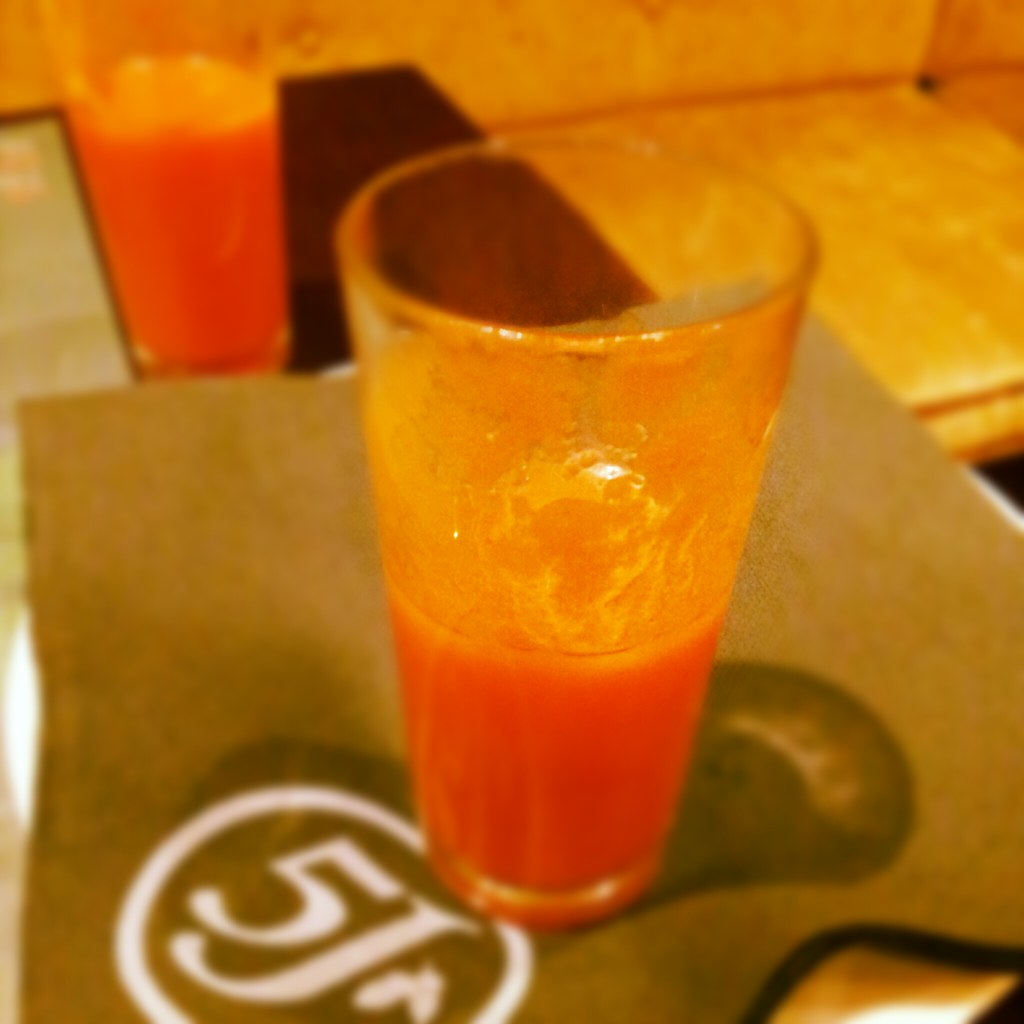This close-up image captures a somewhat blurry, zoomed-in view of a reddish-gold-tinted wooden counter. At the center, a small square-shaped dish holds a shot glass, half-filled with a reddish-orange liquid, possibly a tomato-based or vegetable-based drink. Midway up the glass, there is a yellowish material clinging to the edges. Positioned on an olive green napkin, the dish bears a distinctive white circle featuring the number "5" and the letter "J," accompanied by a logo resembling an upside-down "V." Another identical glass, nearly full of the same liquid, stands behind the dish on the counter. The well-lit area also reveals part of an orange and brown padded wooden bench in the background.